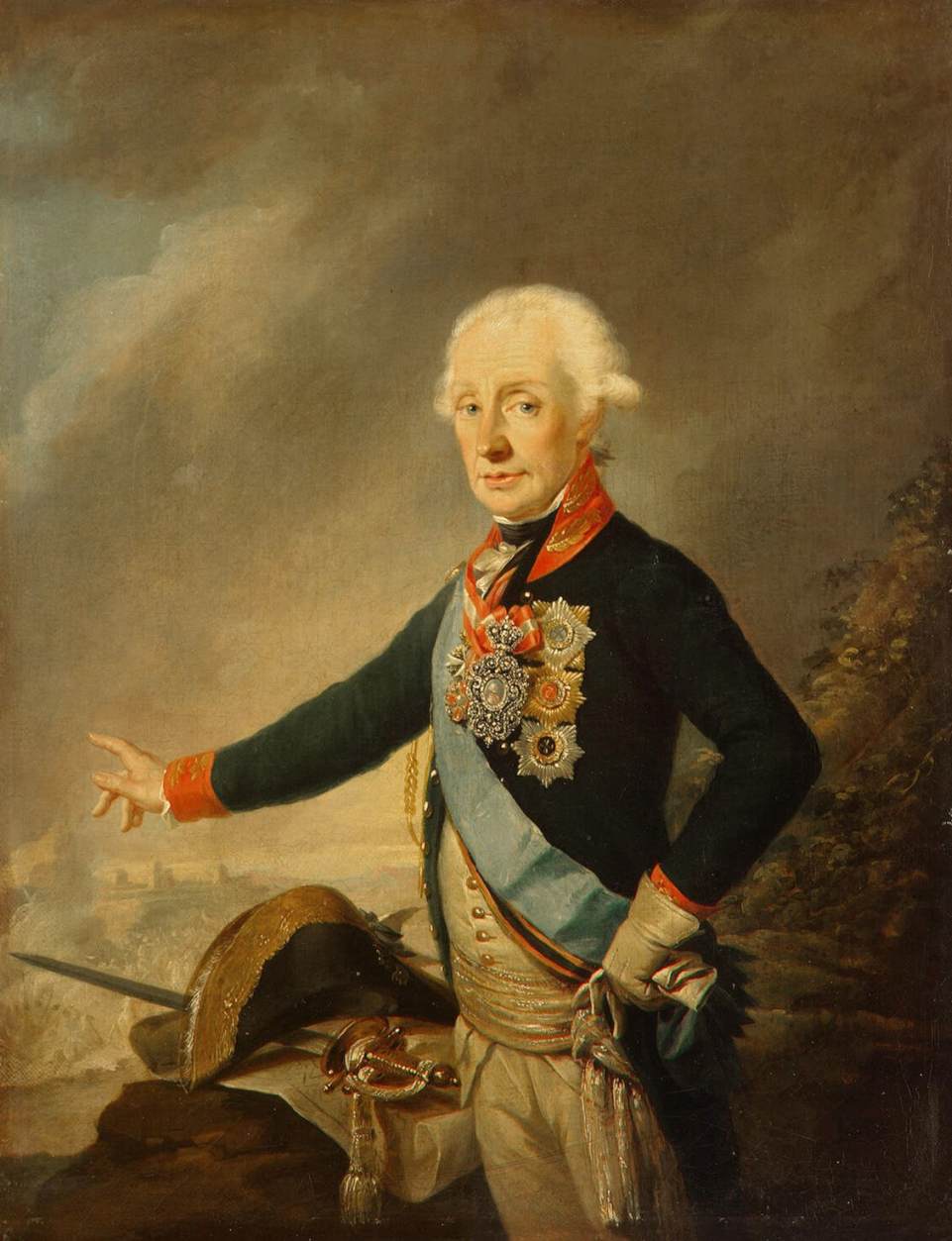This painting depicts an elderly British military officer, evocative of a 1500s or Revolutionary era general. He is wearing a dark uniform adorned with ornate badges and medals, including a brooch with pearls, diamonds, and a crown. His uniform features red cuffs and collar, as well as golden buttons. He has a distinctive white wig, styled short and round, and piercing blue eyes. His right hand, ungloved, points off into the distance, while his left hand, still gloved, holds the right glove. Beneath his black coat, he wears a white shirt and waistcoat paired with white pants and an orange scarf with a gold pattern around his neck. A bluish apron-like garment is also visible around his waist. In front of him, resting on some surface or rock, are his hat, decorated with a pattern, an unsheathed sword, and a paper map. The background is a muted, dark scene with hints of buildings, smoke, foliage, and a grey-brown sky, emphasizing the full color and detail of the central figure.